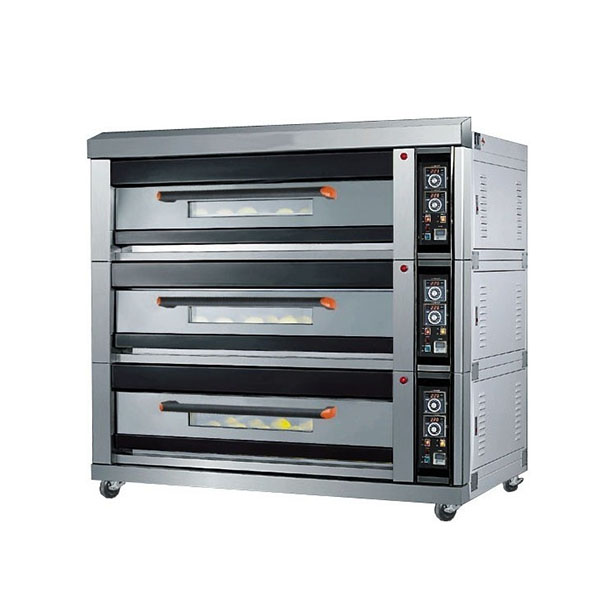The image depicts a three-tier industrial oven, made primarily of stainless steel and designed for a commercial kitchen. Each of the three sections is separated by a solid stainless steel divider and features a drawer with a black metal handle tipped in red, pulling down to access the cooking area. Below each handle is a long, rectangular glass window providing a view into the oven compartments. The oven is mounted on four castor wheels for mobility. Along the right side of the oven, there are various dials and switches to control the temperature and other settings, with each tier having its own dedicated controls. The oven has a sleek, silver appearance with black and red accents, set against a plain white background.